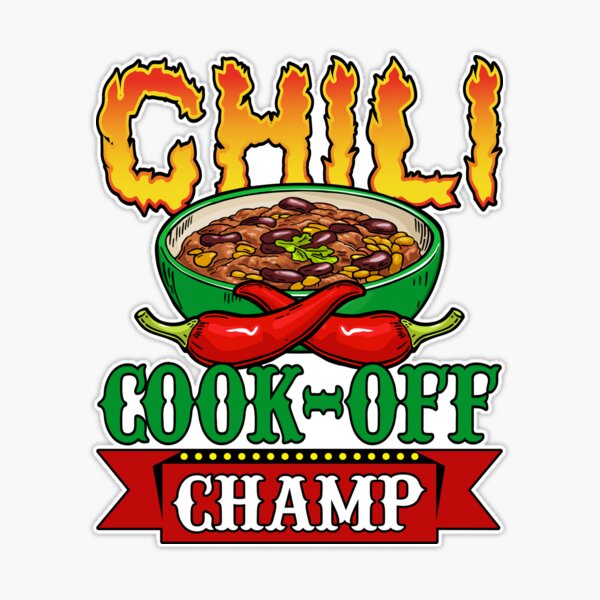The image is a detailed cartoon-style illustration celebrating a chili cook-off champion. The word "Chili" is prominently displayed at the top, crafted to look like flames in red, orange, and yellow hues, symbolizing the spiciness of chili. Below this fiery title, there is a green bowl brimming with hearty chili, featuring brown pinto beans and scattered yellow spots that could be cheese or corn, all topped with a single leaf for garnish. In front of the bowl, two red chili peppers are crossed, adding to the visual interest and spice theme. Towards the bottom of the image, the word "Cook-off" is hyphenated and written in green, followed by the word "Champ" in white text set against a red ribbon background with white dots on a black section resembling lights, emphasizing the celebratory and winning nature of the design. This vibrant and colorful graphic, with its white background, might be used on a t-shirt or similar apparel to proudly showcase someone's victory and prowess in a chili cook-off competition.